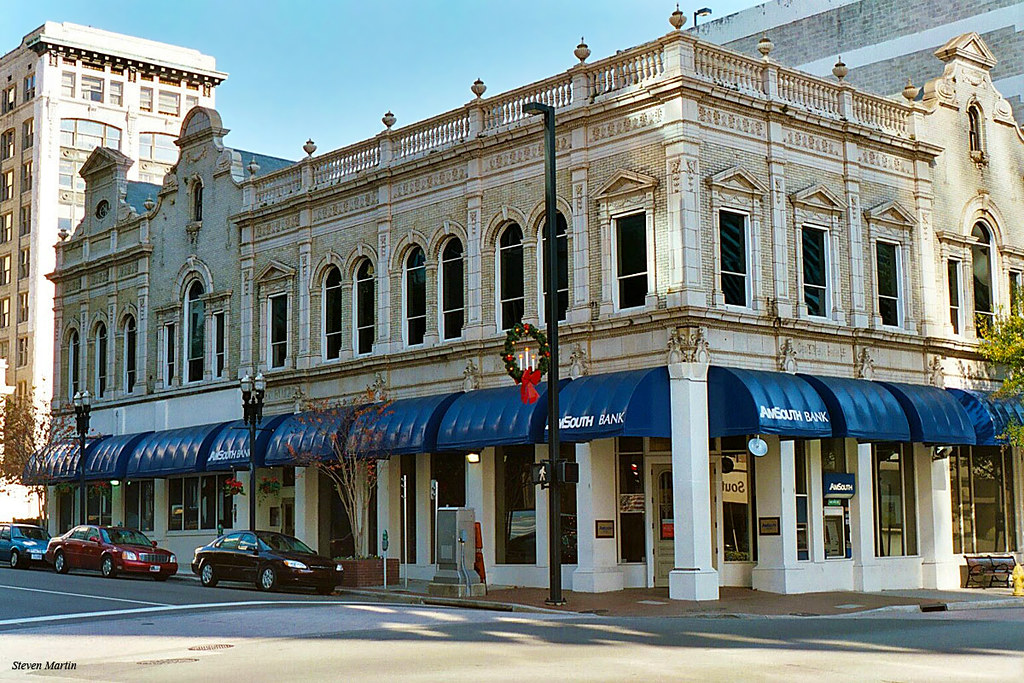In this detailed daytime photograph, we glimpse a beautifully preserved, vintage commercial building, likely over a century old. This two-story, white-brick corner structure boasts European-style, possibly Gothic architecture, accentuated with blue awnings on its multiple entrances. The building functions as a bank, indicated by partial lettering reading "A.N. South Bank" on the awnings. Festive decor adorns the scene, with a green wreath featuring a large red bow and faux candles on a black street pole, suggesting it's Christmas time. The sunny, blue sky casts a warm light over the street, enhancing the nostalgic feel. Three modern cars—black, red, and blue—are parked along the left side of the building, while a yellow fire hydrant and a bench add to the urban charm. The background reveals taller buildings, suggesting a bustling cityscape. Trees are sporadically visible, contributing to the street’s vibrant atmosphere. Lastly, the photo's authenticity is marked by the name "Steve Martin" printed at the bottom.